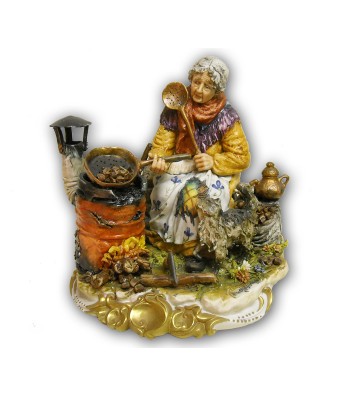The image depicts a detailed ceramic figurine of an elderly woman, adorned in a white mob cap, a yellow sweater, a purple shawl, an orange scarf, and a flowered skirt with a hole revealing her knee, clad in yellow and green tights. She appears to be seated on a rock formation, engaged in cooking over a small, battered burning barrel with visible flames. In her right hand, she holds a frying pan over the fire, while her left hand rests a large covered ladle on her right shoulder. Surrounding her are various kitchen and camping tools, including a lantern on her left and a teapot on a stump to her right. The scene is accentuated by a woodland and grassy environment underneath her feet, making this well-painted, small figurine a charming display piece, possibly suitable for a kitchen.